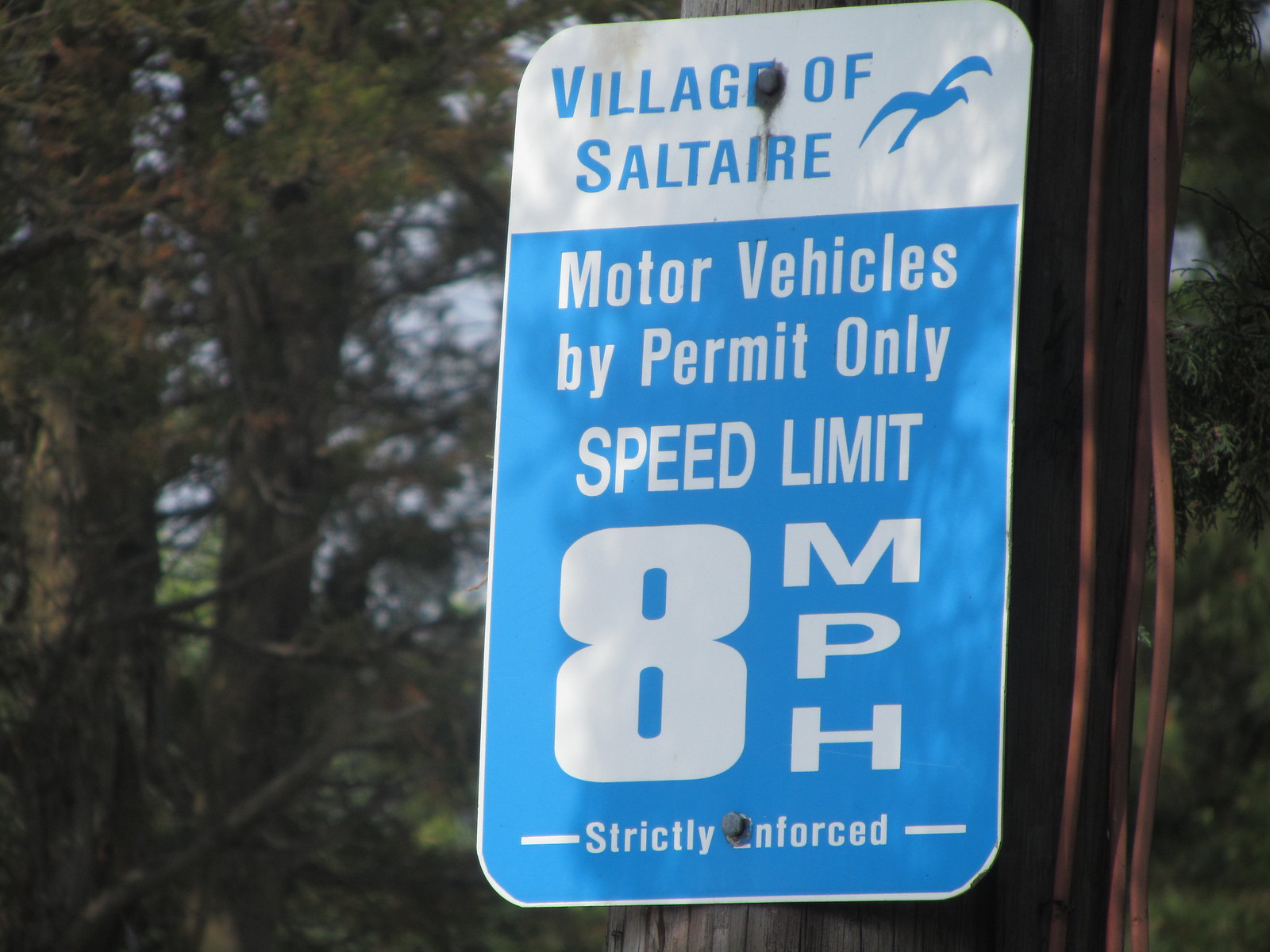The image features a light blue and white speed limit sign prominently displaying "Village of Salterre" at the top in blue text, accompanied by a blue silhouette of a seagull. Below this, the sign specifies "Motor Vehicles by Permit Only" and clearly states a "Speed Limit 8 Miles Per Hour," noting that this regulation is "strictly enforced." The large white number eight is particularly noticeable. The sign itself appears to be bolted to a brown, wooden pole reminiscent of a telephone pole. Surrounding the sign, a blur effect suggests a backdrop of large, light green trees under a bright, sunny sky. Additionally, some wires can be seen draped down to the right of the sign.